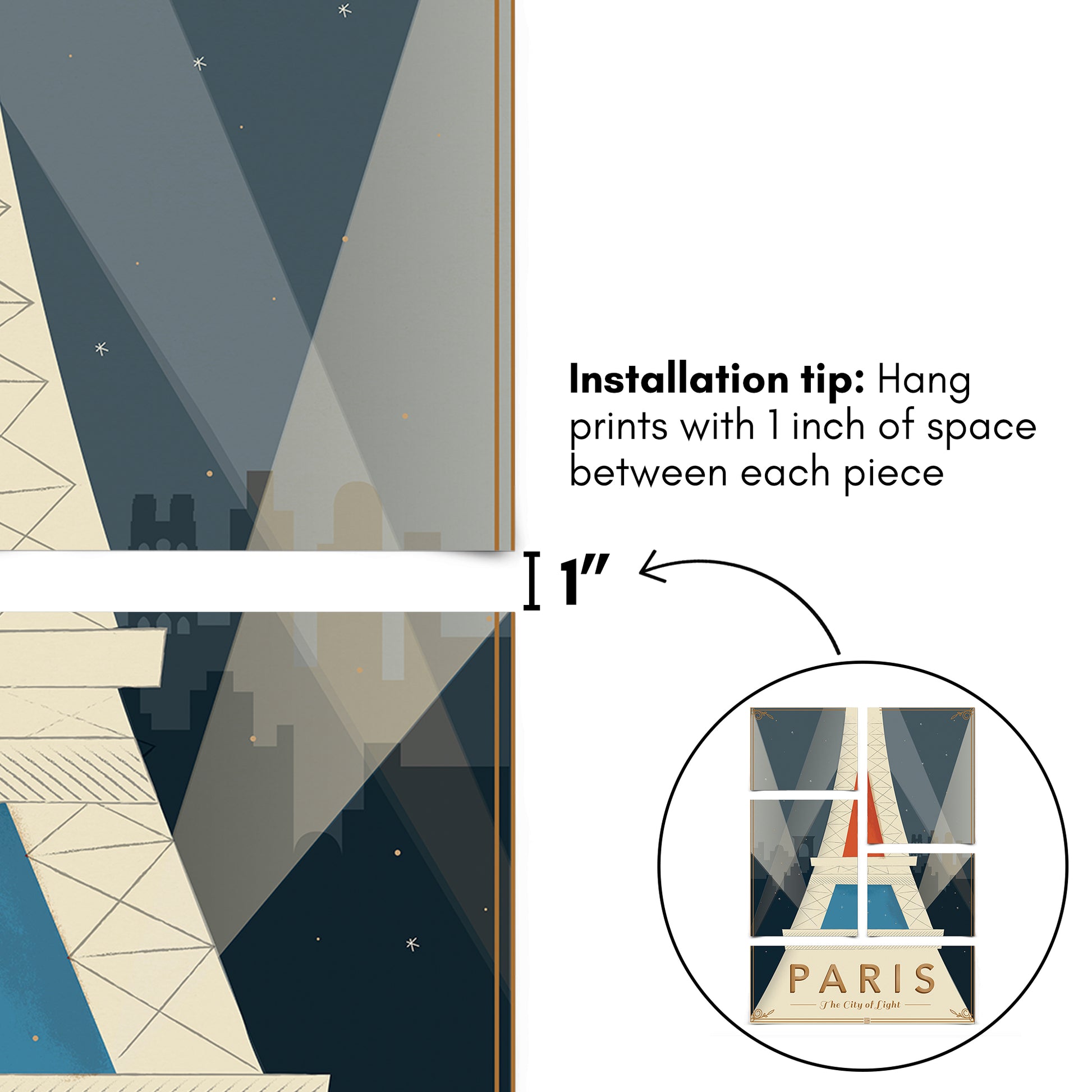This image is a detailed poster providing instructions on how to hang a multi-part print of the Eiffel Tower for optimal visual appeal. The primary focus is on five pictures of Paris, specifically depicting the Eiffel Tower within a circle at the bottom right of the layout. The Eiffel Tower print is simplistic with white and gray or blue markings, representing the metal structure. Beneath this image, the word "Paris" is prominently displayed in yellow, followed by the text "the city of light."

On the top left of the poster, there are two separate square areas. The first square area shows a starry sky with tall building silhouettes in a simplistic drawing style, featuring a diagonal light gray section. This gray section extends into the second square below, where it angles more towards the bottom middle, showing additional buildings and a few stars.

Adjacent to these squares, the poster includes an installation tip in black text: "Hang prints with one inch of space between each piece," which is repeated on the right side of the poster over a white background. This instruction is exemplified by the depicted layout with a one-inch gap between the prints. An arrow from the circle points to this exemplary arrangement, emphasizing the suggested spacing for a cleaner and more organized presentation.